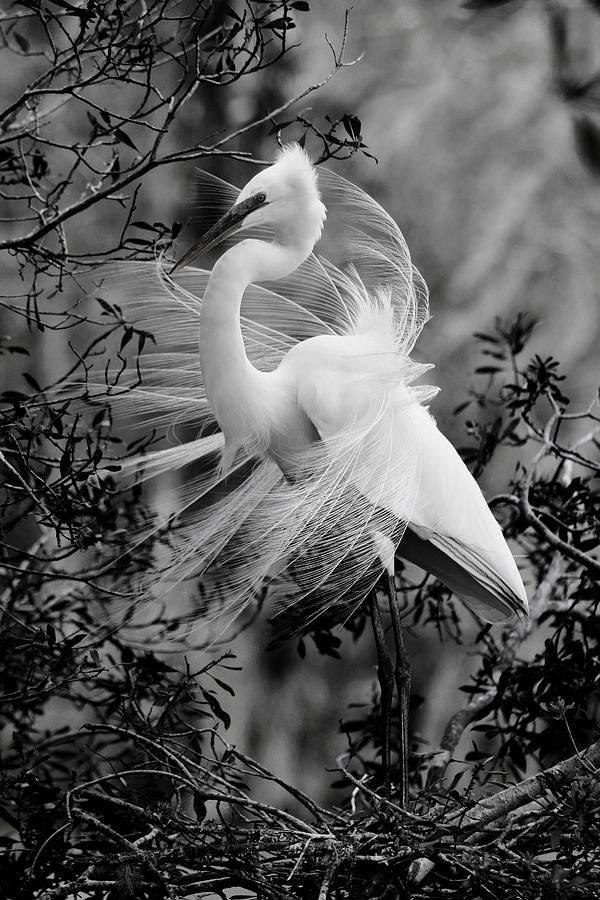This high-resolution, black-and-white photograph captures the essence of art photography with its finely composed depiction of a snowy egret, a majestic water bird renowned for its elegance. The egret, with its long, slender legs and elongated white neck, stands poised on what appears to be a nest made of twigs, nestled within the branches of a tree or bush. Its sharp, dark beak is pointed and ready for fishing, a characteristic feature of its species. The scene is tranquil yet dynamic, as a gentle breeze ruffles the egret's wispy, gauzy tail feathers, blowing them forward across its body, enhancing the bird's graceful appearance. The background is skillfully blurred, with only hints of leaves and flowers framing the egret, drawing focus to its exquisite form and serene posture. The delicate interplay of the bird's white plumage against the subdued backdrop creates a striking contrast, making this image a captivating portrayal of wildlife in its natural elegance.